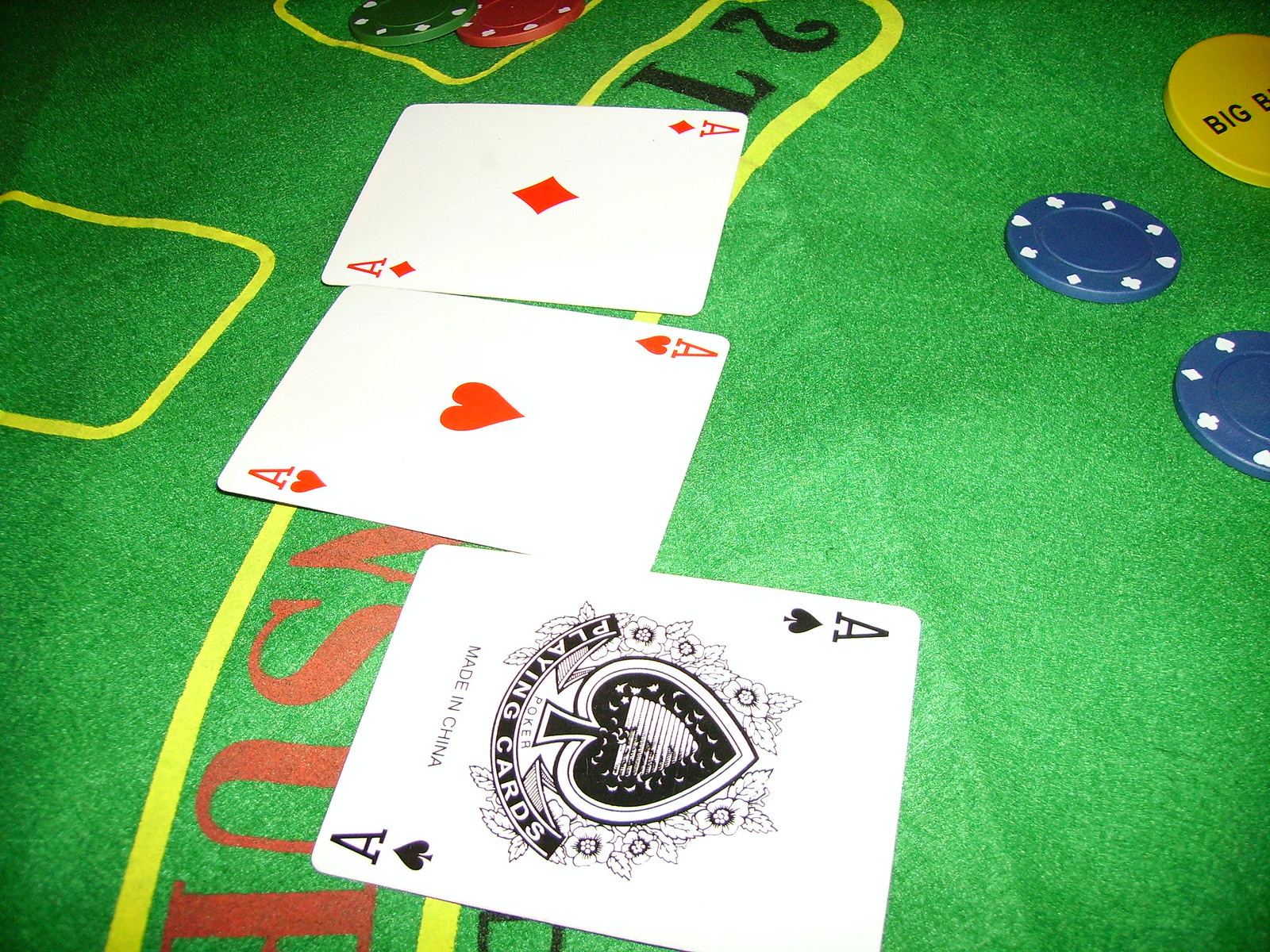The image features a predominantly green background with a subtle gradient, becoming darker towards the upper left corner. On the left side, there are two yellow-outlined squares with rounded corners; one is positioned near the center and the other near the top. Both squares have green interiors. The upper square contains two poker chips: one green with white dots and one red with white dots. Below these, there is a long yellow-outlined, curved shape with a green center. At the top of this shape, "2T" is written in black. The bottom part holds red writing, though it is obscured by a fan of playing cards. The cards displayed are an Ace of Diamonds, followed by an Ace of Hearts, and an Ace of Spades at the bottom. On the right side of the image, two blue poker chips with white dots are visible. Additionally, in the upper right-hand corner, there is a segmented yellow circle with the partially visible word "BIG" and the letter "P," with the rest of the text cut off at the edge of the picture.